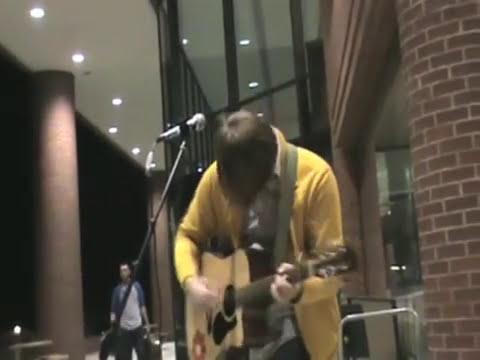This image captures a detailed interior scene, possibly a high school auditorium or concert hall. Prominent in the foreground, a man with brown hair plays an acoustic guitar. He's wearing a yellow cardigan with a white collared shirt underneath, and his head is bowed, hiding his face with his hair. The guitar is strapped over his shoulder, and he stands next to a microphone on a stand. Surrounding him, a tall brick column stands to the right near a large plate glass window, possibly two stories high, reflecting recessed ceiling lights. To the left, more brick columns support a white ceiling with can lights illuminating the scene. In the background, slightly shrouded in darkness, another man is visible with a white shirt with blue sleeves, holding a couple of bags. The composition of pillars, an awning-like structure, and the ambient lighting suggests it's evening or night inside this spacious interior setting.